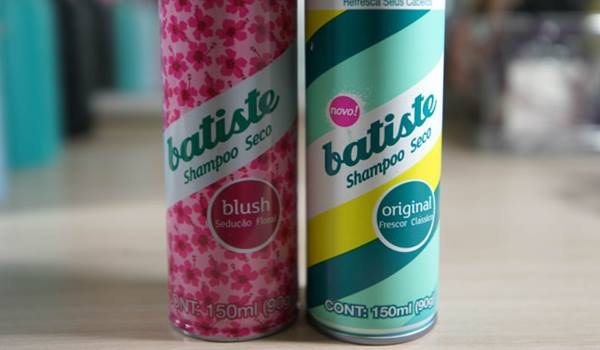In the center of the image, there are two tall, skinny cans positioned on a smooth surface, which could be a counter or the floor. The background is blurry, making it hard to discern additional details, but the setting suggests it could be someone's home or a store that sells the products. The can on the left is labeled "Batiste Shampoo Seco Blush" and features pink and red flower designs. The can on the right is labeled "Batiste Shampoo Seco Original" and has light blue, light green, dark green, and yellow stripes. Both cans contain 150 milliliters, which is equivalent to 90 grams. The predominant colors in the image include blue, pink, red, purple, white, and pale hues.